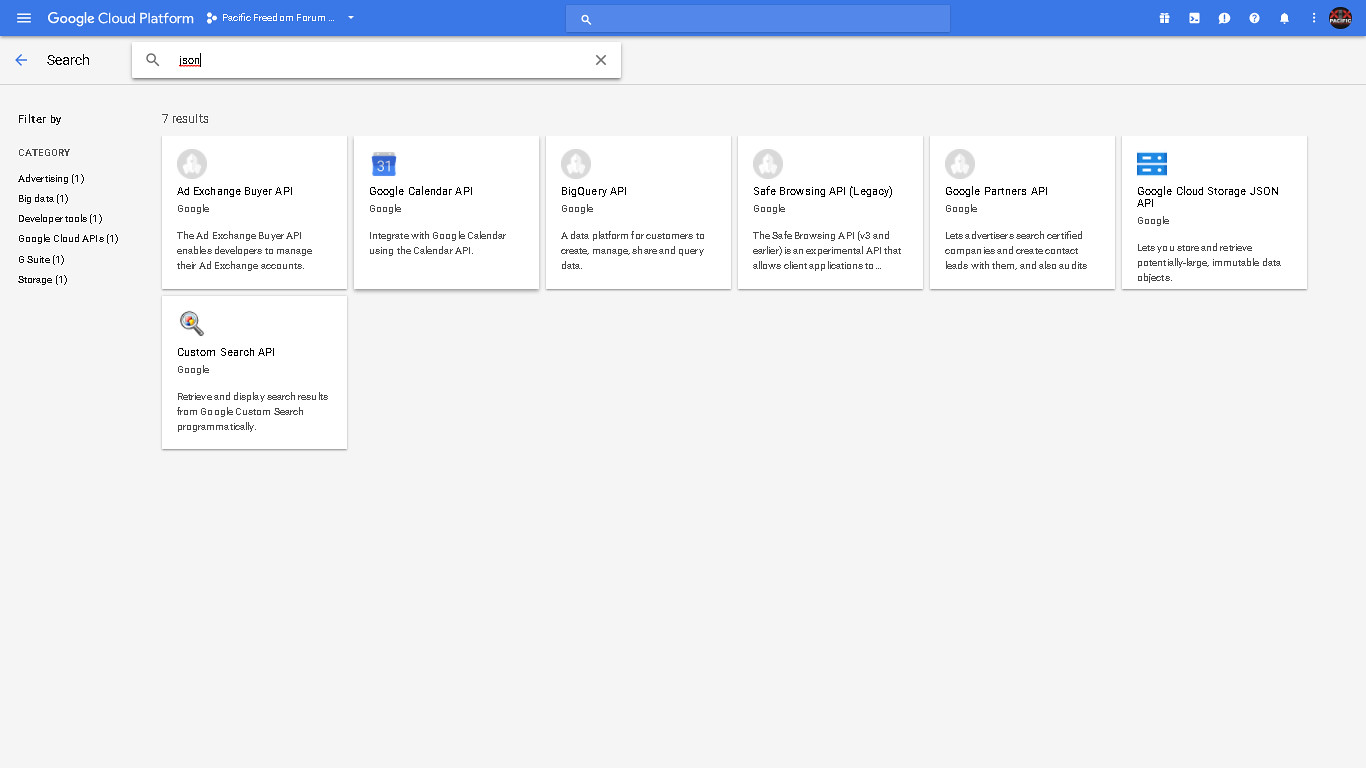The image is a detailed depiction of the Google Cloud Platform interface in a rectangular format extending from left to right. The top portion features a blue strip with the "Google Cloud Platform" logo in white text, accompanied by three parallel lines. Beneath this, there's a smaller text in white, the content of which is unclear. A white search bar with a magnifying glass icon is prominently displayed, allowing users to enter text. On the left side of the search bar, there are several white icons, including a set of three dots and another image icon.

Below this blue section, the interface transitions into a gray strip followed by another white strip containing a similar search bar, already populated with partial text that appears to start with "I" or "In". Adjacent to the search bar is a gray 'X' icon for clearing the search input. 

Underneath the search bar is a filter section labeled "Filter by" in black text, listing various categories such as "advertisement," "big data," "developer tools," "Google Cloud APIs," "G Suite," and "storage," alongside a count of seven results in black text.

The lower section of the interface is divided into grids of light gray square boxes. The first row contains six boxes, each displaying an icon followed by the title in black text and a brief description. The second row includes just one box, maintaining the same format of icon, title, and description.